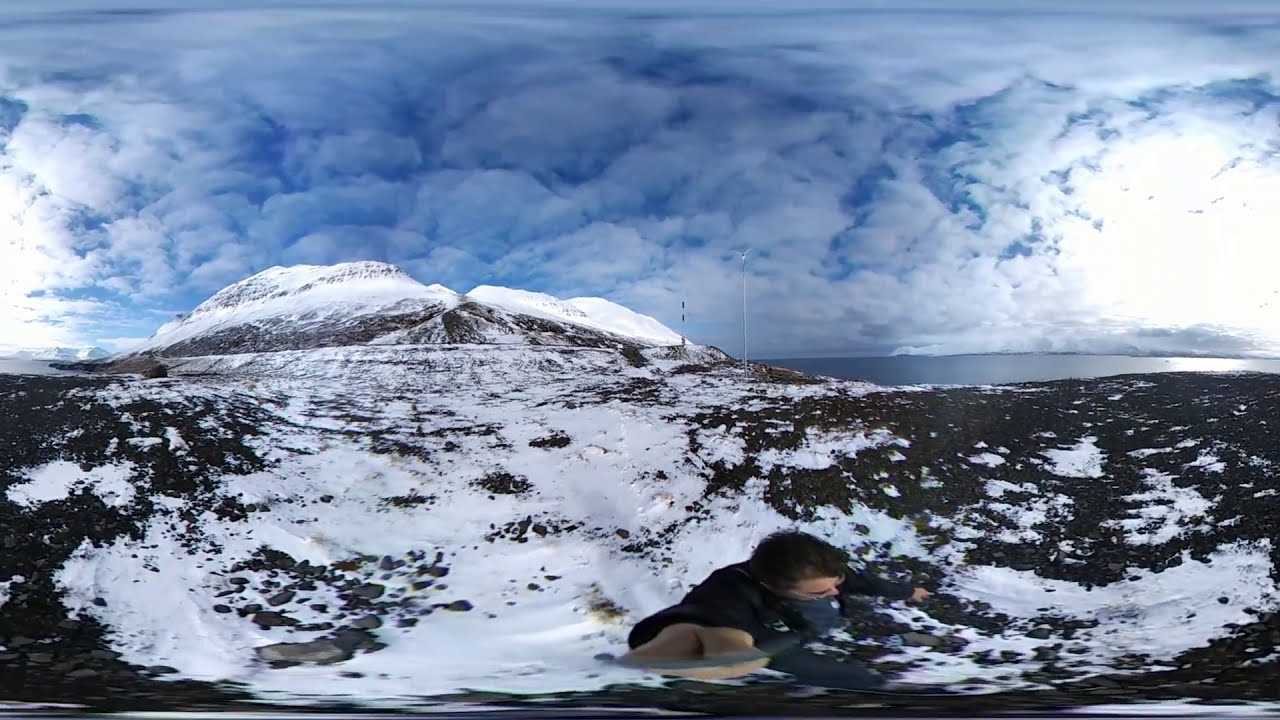This horizontally aligned rectangular photo, seemingly taken with a fisheye lens, captures a visually engaging snowy mountain landscape. Dominating the center-left of the image is a majestic snow-capped mountain with jagged black rocks interspersed with patches of snow. In front of the mountain, there's lower-lying land partially covered with snow and rock.

The sky above is beautifully adorned with layers of fluffy, feathery white clouds against a blue backdrop, with particularly bright white areas on the far left and right sides. Towards the center-right, there is a body of water that adds to the scenic outdoor setting.

At the bottom right of the photograph, there's a man with short brown hair, dressed in a black long-sleeve shirt or dark-colored jacket. He is crouched or kneeling down, with his right arm extended towards the viewer and pointing to the left. The bottom portion of the image, including his legs and right hand, appears somewhat distorted, likely due to the lens effect, curving outwards and affecting the overall perspective. This distortion gives the photo a unique, almost surreal quality.